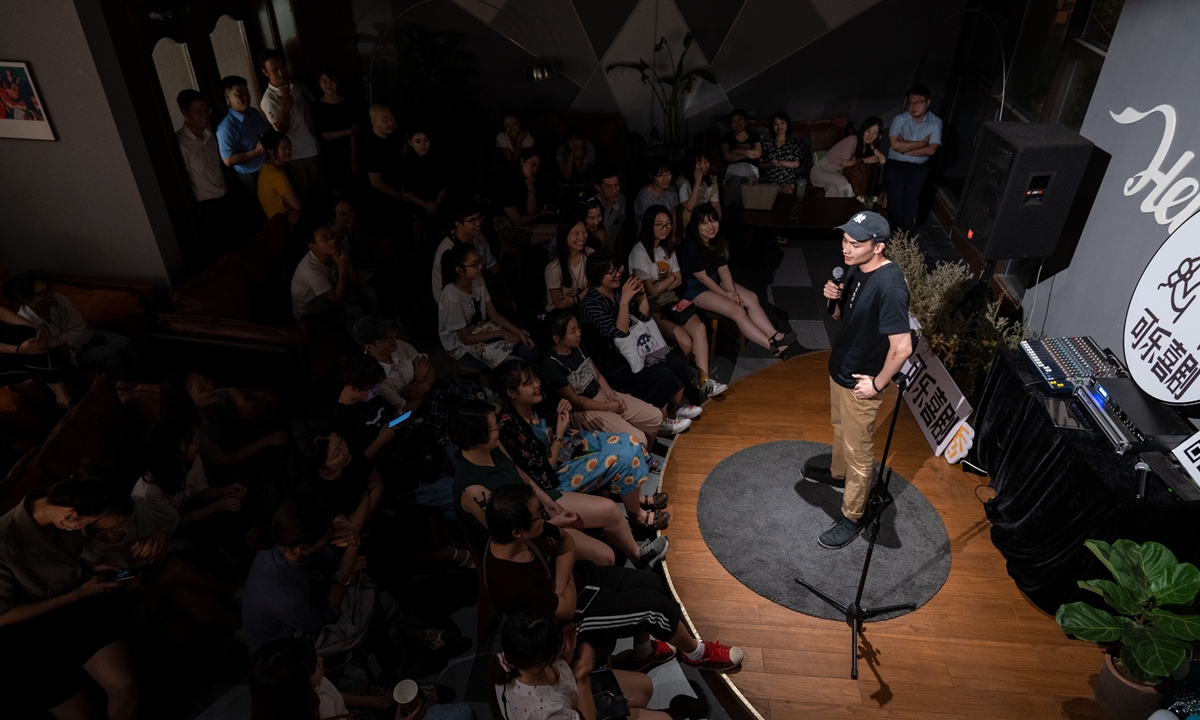The photograph offers a bird’s-eye view of a cozy, semicircular stage crafted from polished wood. Bathed in spotlight, an Asian comedian stands center stage, distinguished by his black baseball cap, black t-shirt, khaki pants, and black shoes. With a microphone held to his face, he captivates the audience clustered around him in the dimly lit foreground. Behind him, technical equipment and a mic stand hint at the performance setup, while signs with Asian characters, possibly Chinese or Japanese, frame the scene. The audience, predominantly young and Asian, sits tightly packed around the stage, their presence fading into the darkness beyond the illuminated performer.